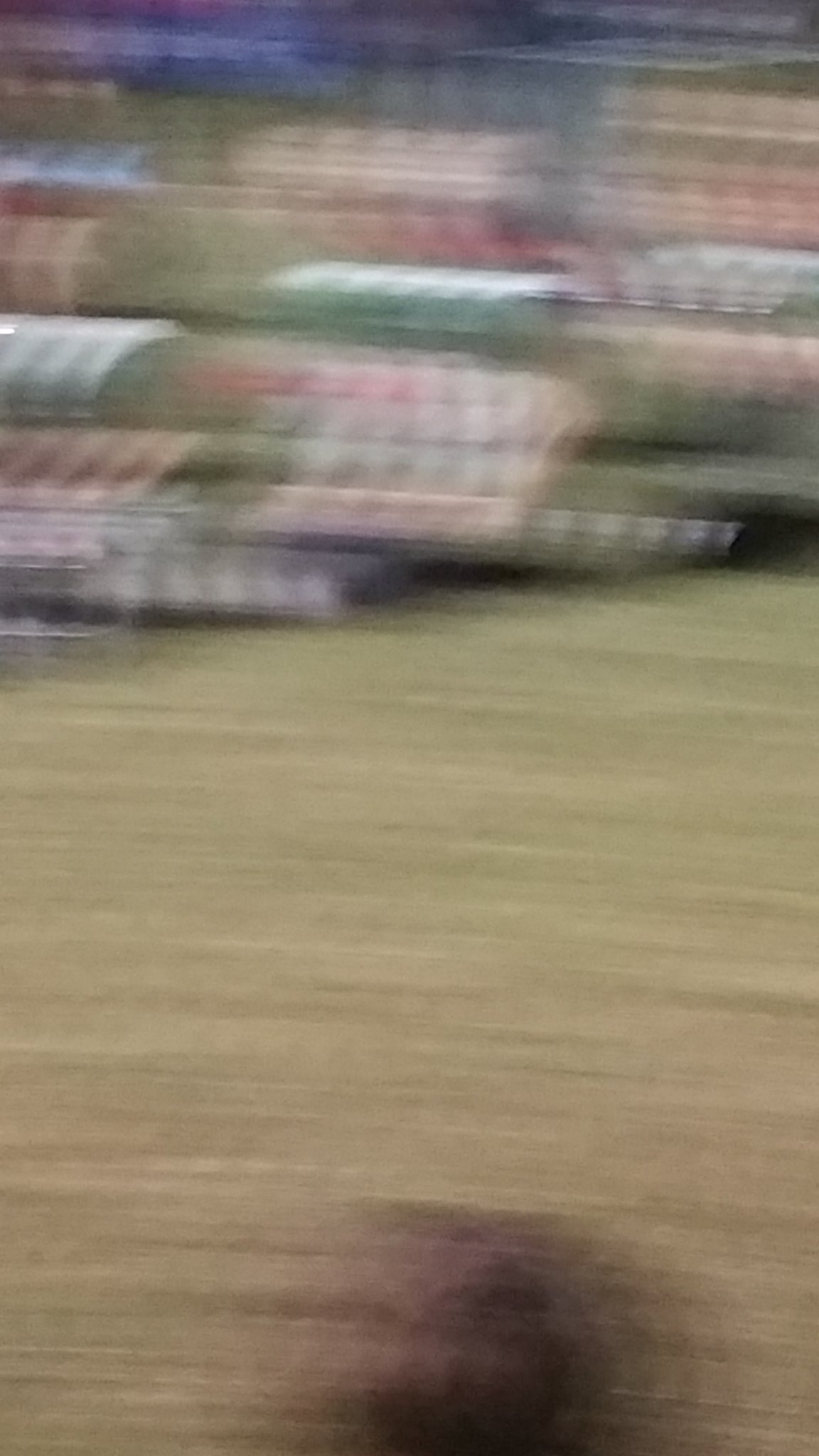The photograph, taken in portrait orientation, is extremely blurry, suggesting it was captured at a high speed, possibly from a moving vehicle like a car or train. The image features a vibrant mix of colors: red, green, dark blue at the top, and various light and dark shades towards the bottom. It depicts a landscape that includes grassy areas and light-colored ground with a dark bottom section. 

At the very bottom center, there's a barely discernible dark, blurry figure resembling a human shape. The image is mostly characterized by blurred streaks of green, yellow, and light brown, possibly representing a pasture or grassy field. Towards the top, there appear to be multicolored objects—potentially rooftops or stacked items—in hues of green, pink, blue, red, and white, all blending together in an indistinct, streaked manner. The photograph's overall impression is chaotic and colorful, with horizontal and vertical blur lines suggesting it was taken during quick motion, making it difficult to identify specific details clearly.